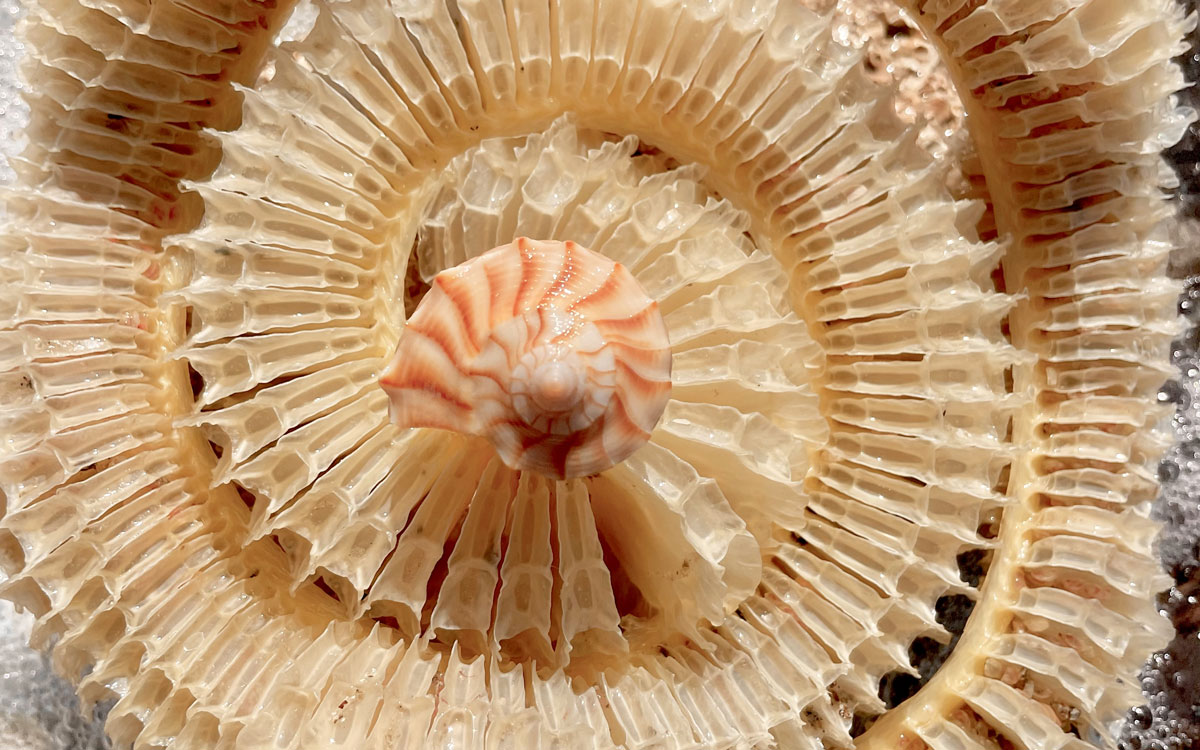In the center of the photograph, there is a cream-colored conch shell adorned with orange stripes that spiral inwards, resembling the shape of a crescent roll. The shell features distinctive ripples and culminates in a small, rounded point at its tip. This conch shell is perched on top of a much larger and intricately detailed spiral structure. The underlying structure, possibly a fragment of another shell or a skeleton, exhibits a ribbed or spiny texture, reminiscent of a honeycomb pattern. The myriad of small, spiked sections form a continuous, ornate swirl around the central shell, creating a visually captivating and elegant composition. Surrounding the intricate arrangement are bubbles, indicating that the scene could either be on the sea floor or floating in water.